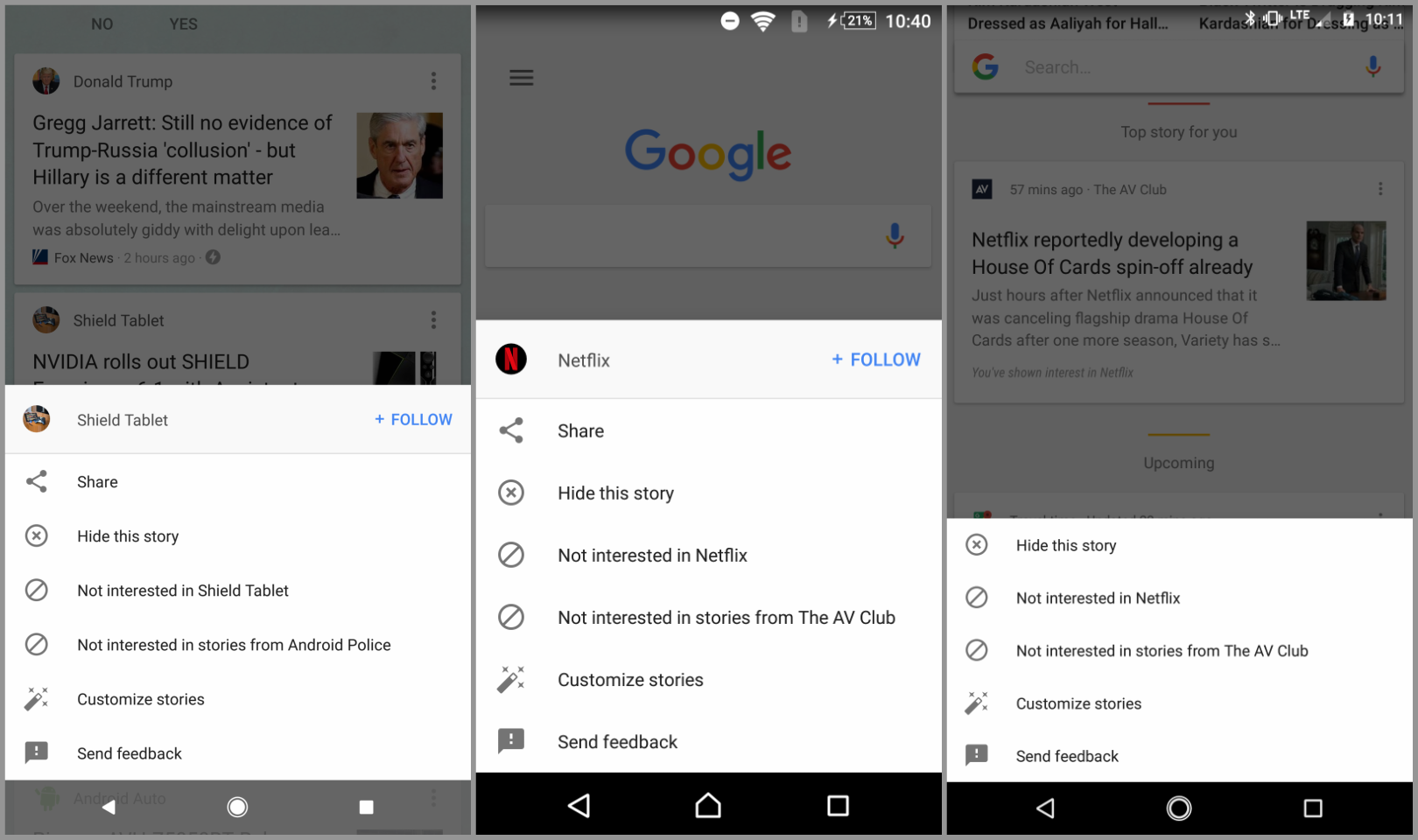In this image, we see three distinct smartphones, each displaying different webpages. Starting from the left, the first phone features an illuminated triangle, circle, and square at the bottom of its screen. This phone also has a dark gray bezel. The screen shows a Google News feed with a grouping of suggestions, including a profile picture and the name "Shield Tablet," along with options like "Follow," "Share," "Hide this story," "Not interested in Shield Tablet," "Not interested in stories from Android Police," "Customize stories," and "Send feedback."

In the middle, the second phone has a black bezel and is showing just the Google search bar with the Google logo. Below the search bar, it features a news snippet about Netflix with an option to follow it. The options are similar to the first phone, including "Share," "Hide this story," "Not interested in Netflix," "Not interested in stories from AV Club," "Customize stories," and "Send feedback."

The third phone on the right, also with a black bezel, displays an aggregated Google News page. At the top, partly obscured, it shows "dressed as ANLIYAH4HALL" and an incomplete name. The menu options on this screen include "Hide this story" with an 'X,' "Not interested in Netflix," "Not interested in stories by AV Club," "Customize stories," and "Send feedback."

Each phone displays different content and menu options, illustrating various configurations and news interests on the Google News platform.